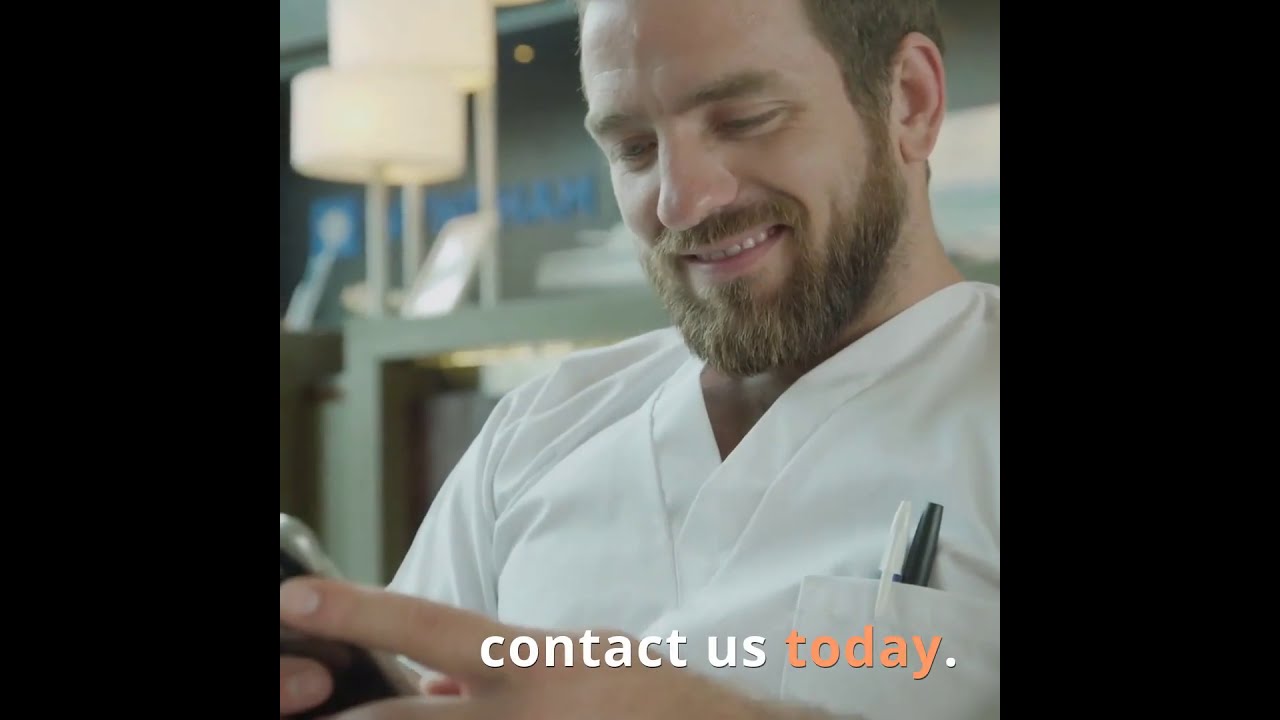The image features a close-up of a white male with reddish-orange hair and beard, smiling as he looks down at his phone, seemingly texting or viewing something on the screen. He is wearing white v-neck scrubs with a chest pocket that contains two pens, one black and one white. The top of his head is cropped out of the picture, but his expressive features, including thick eyebrows, are visible. The background includes two tall, blurry lamps emitting a yellowish-white light and a wall with some blue writing on it. On both the left and right sides of the image are solid black vertical bars. At the bottom right of the image, white text reads "Contact us," and in orange, "today" with a period, completing the message.